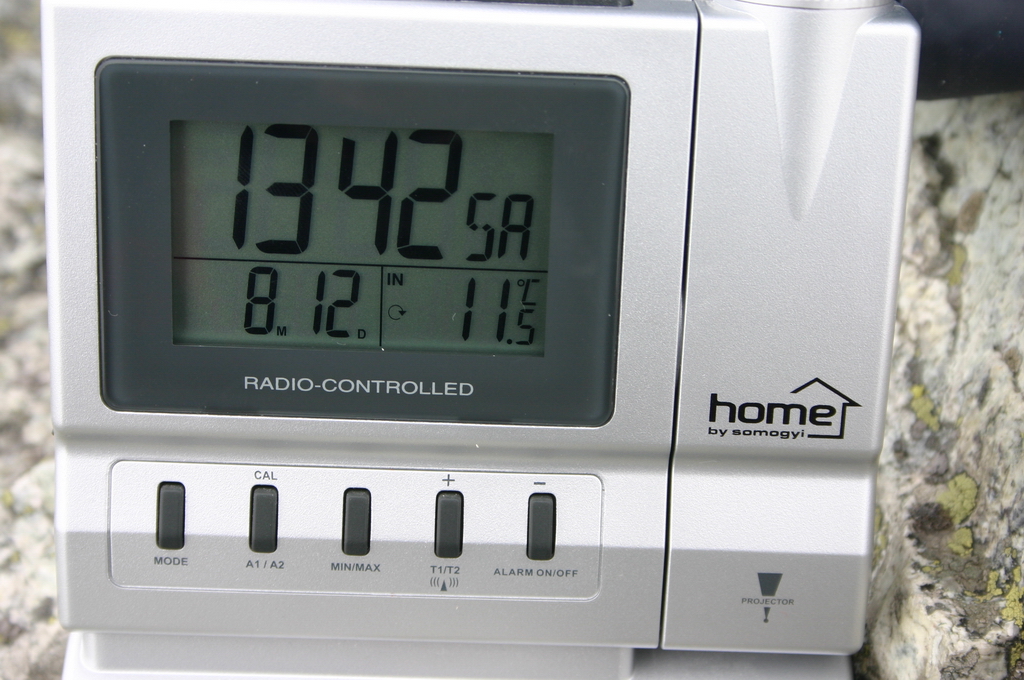The image appears to depict a digital thermostat, likely used for controlling the heating and cooling system within a household. The device features a sleek, white casing with a gray interior border surrounding its display. The screen is an LCD type, showcasing clear black lettering and numbers against a light background. The display includes crucial information such as the current time and date, showcasing them prominently for easy readability. Temperature settings are shown in Celsius, indicating the current indoor climate conditions, and the thermostat is labeled as "Radio Controlled," suggesting it may sync its time and settings wirelessly for accuracy. Additionally, the thermostat is branded with "Home by Energy," hinting at the manufacturer or product line. Control buttons, also black, are situated below the display for user interaction. Overall, this thermostat combines functionality with a user-friendly interface for efficient home climate management.